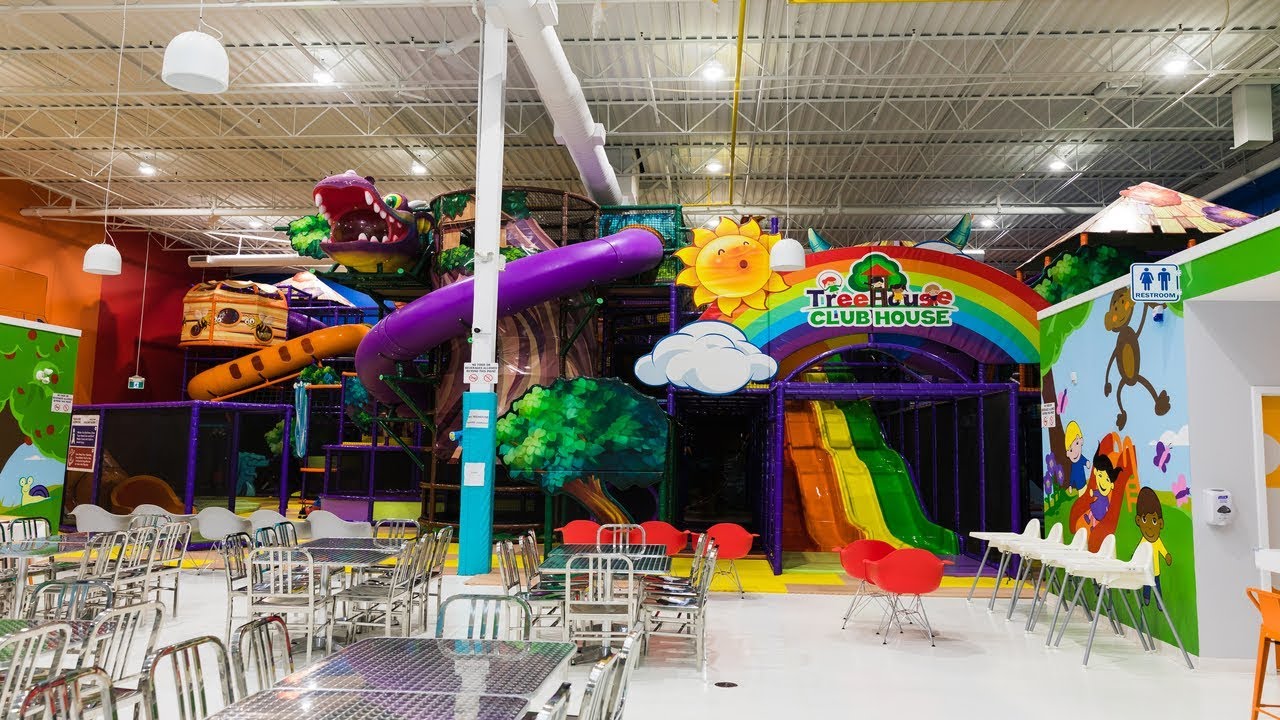The image showcases a vibrant indoor entertainment center called "Treehouse Clubhouse." Situated inside what appears to be a warehouse with an industrial ceiling featuring exposed pipes, framework, and lights, the setting is both functional and playful. The smooth white concrete floor extends throughout the space, contrasting with the colorful attractions.

At the heart of the clubhouse is a large mural and logo that reads "Treehouse Clubhouse," crowned by a rainbow arch. Beneath the arch are four multi-colored slides - red, orange, yellow, and green - that enhance the playful theme. To the side of these, a large tunnel slide with a distinctive alligator face can be seen, adding to the amusement park-like atmosphere.

The surroundings are filled with child-friendly decorations, including murals of cartoon characters like monkeys and playful children, and a restroom area with painted frogs and kids. The foreground is populated with clusters of red and white metal chairs arranged around tables, providing ample seating for visitors. Additional play areas for children are also present on the left-hand side of the venue, making it a comprehensive indoor playground designed for special events and entertaining young guests.